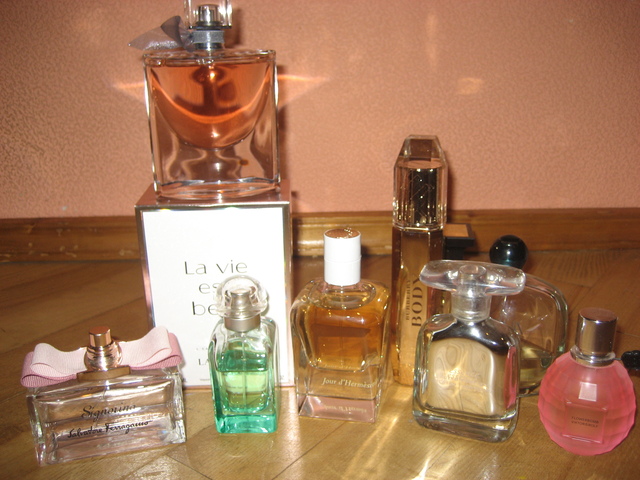In the photograph, a collection of approximately eight meticulously arranged perfume bottles is displayed on a wooden floor. The background features peach-toned walls and a wooden baseboard, adding a warm ambiance to the scene. The bottles vary in shape, size, and color, offering a visually appealing and diverse array. 

Starting from the left, there is a short, wide rectangular bottle with a clear liquid inside, adorned with a pink ribbon and a gold atomizer. The text on it reads "Signorina" by Salvatore Ferragamo. Next to it is a taller, slender bottle containing clear blue liquid. Following is a larger, square bottle with a white cylindrical cap, though the text on it is unreadable. Further to the right, there is a rectangular bottle with a T-shaped stopper. On the far right is a round, pink bottle resembling a globe or grenade, with a ridged design and a silver metal top.

In the background, three additional bottles add depth to the arrangement: one with a more rounded shape and a green spherical stopper, another gold-colored bottle inscribed with "Burberry Body," and a tall bottle with pink liquid and a silver ribbon encased in a white box with a silver outline, labeled "La Vie est Belle."

The bright lighting accentuates the reflections and intricate details of the glass bottles, creating a captivating and detailed visual experience.